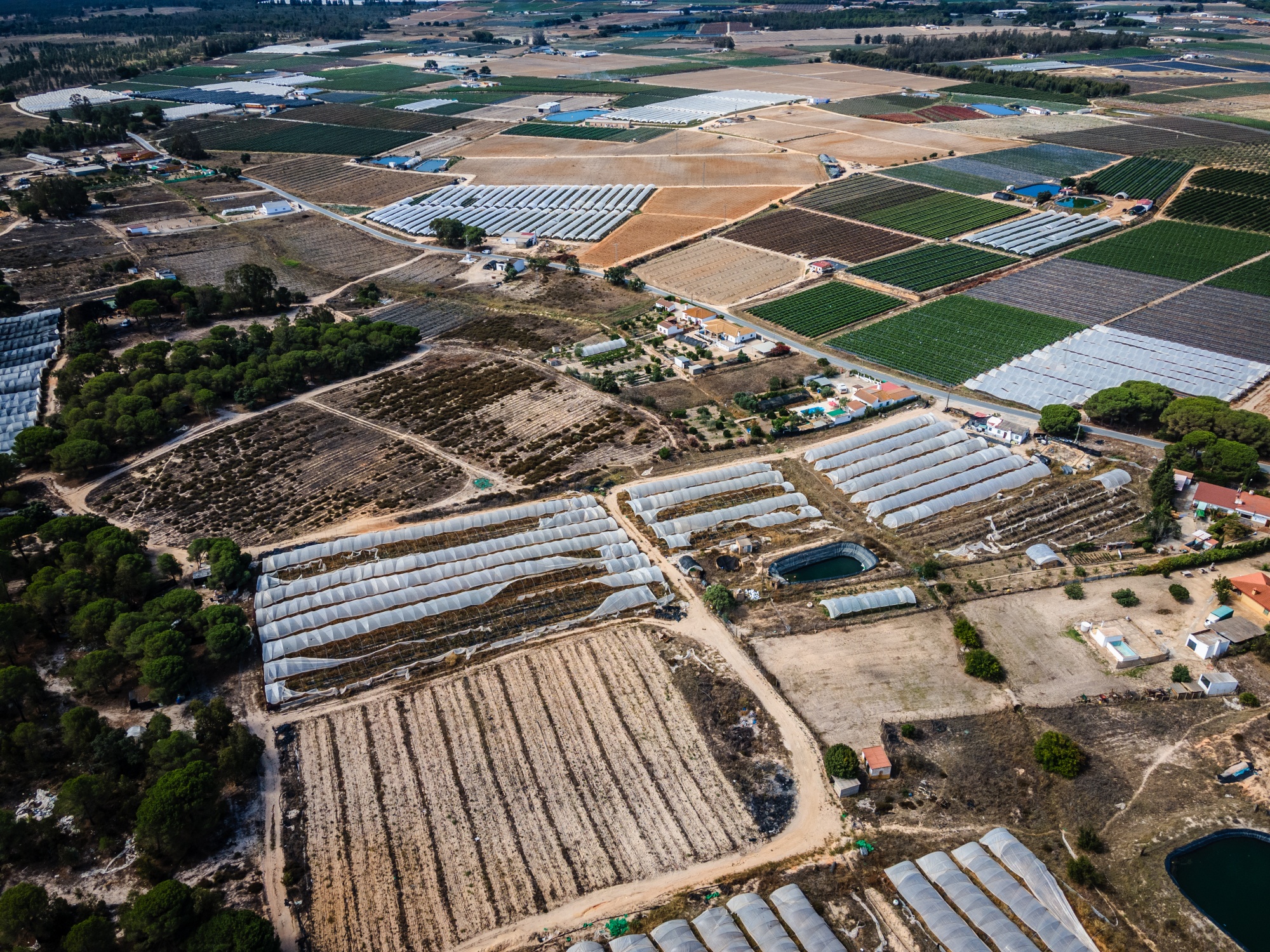This aerial photograph captures an extensive, parceled landscape that appears to be a farming community comprising several acres. The fields are meticulously divided into various sections with distinct visual features. Dominant throughout the image are long strips of land, some covered with white plastic, which likely serves to protect rows of crops, seeds, or possibly hay bales. These plastic-covered rows are interspersed with areas of light brown fields, suggesting that crops have recently been harvested. There are diverse patches of earth, ranging from light to dark brown, indicating different soil preparations or stages of planting. Scattered across the landscape are clusters of buildings, including houses and long barns, hinting at a blend of residential and agricultural infrastructure.

In the distance, the pattern continues with more parceled sections, some of which are not yet planted while others are similarly covered with protective plastic. The landscape is also punctuated by small clusters of trees and water features, likely ponds, which add to the diverse agricultural environment. The fields exhibit various hues of green, brown, and tan, reflecting different types of crops and growth stages. This photograph, devoid of any specific geographic indicators, provides a detailed and intricate view of an agricultural endeavor marked by human organization and varied land use.